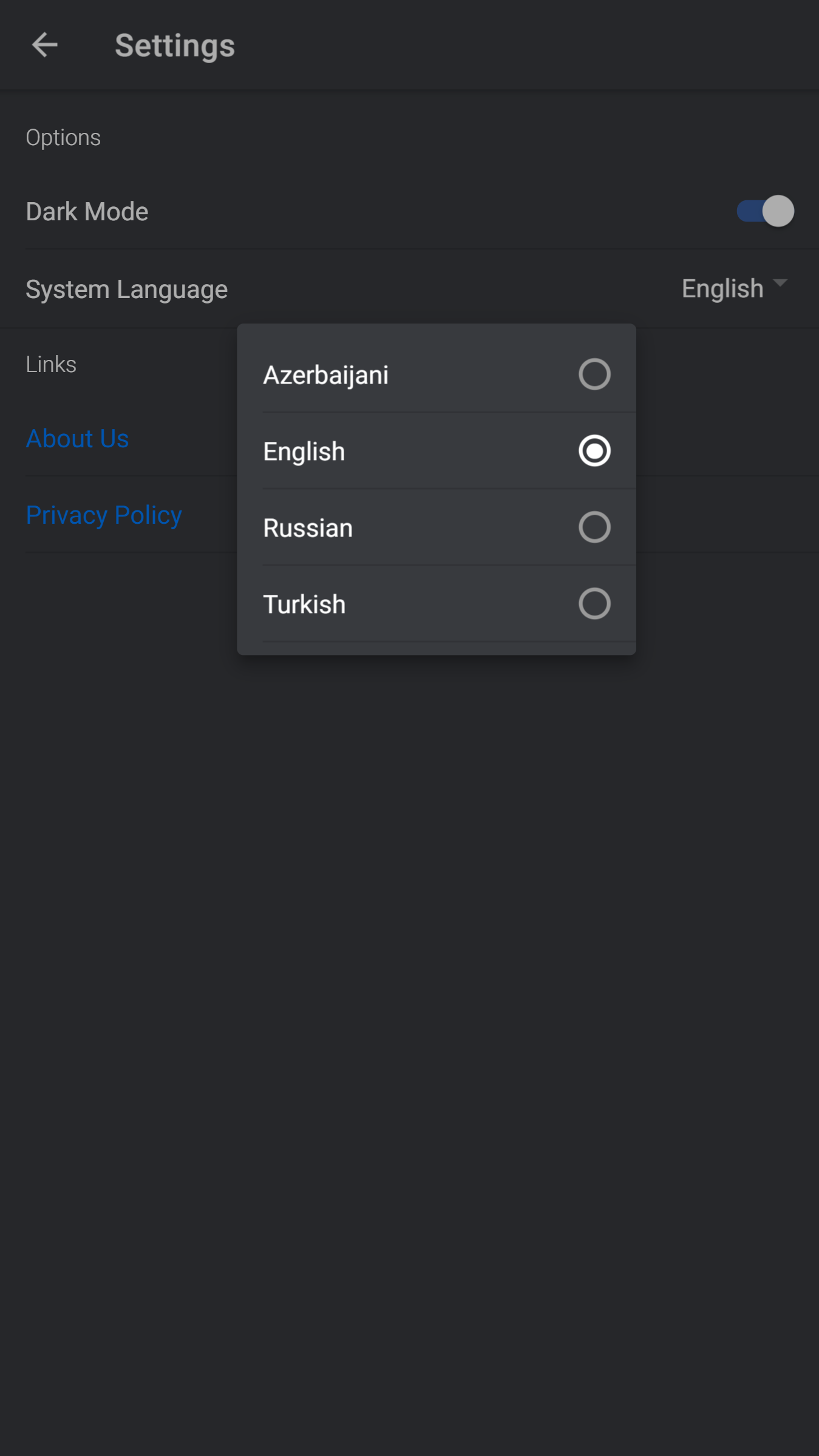This vertical screenshot features a predominantly dark gray theme indicative of an activated Dark Mode. At the very top, a back or left-facing arrow is visible, allowing navigation to the previous menu, signaling that we are currently in the settings section. 

The title "Settings" is displayed in white text against the dark gray background, followed by a subsection labeled "Options." Below this, the text "Dark Mode" is clearly marked and actively enabled, highlighted by a blue toggle indicator.

Further down, the "System Language" setting is presented with a drop-down menu. This menu currently shows four language options: Azerbaijani, English, Russian, and Turkish. The second option, English, is selected, as evidenced by the white filled-in circle next to it, with the drop-down box prominently positioned in the middle of the screen.

Below the system language section, there is a segment labeled "Links," also in white text. Under this segment, clickable sections for "About Us" and "Privacy Policy" are visible, distinguished by their blue text, indicating that users can interact with these links.